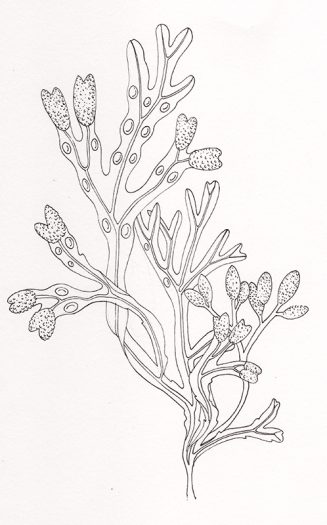This black-and-white sketch features a central tree limb extending vertically from the bottom to the top of the image. The limb is intricately detailed with multiple branches and stems sprouting off in various directions. At the tips of these branches and stems, there are numerous flowers depicted in different stages of blooming. Some flowers are heart-shaped, while others have an oval, spoon-like appearance. Delicate veins are visible running through the stems, adding to the intricate detail. The entire composition is set against an all-white background, emphasizing the stark contrast of the black sketch lines. This detailed drawing captures the natural beauty and complexity of a flowering tree limb, with no text or additional elements to distract from the artwork.